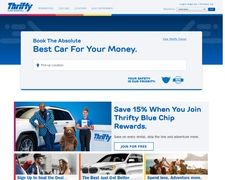On the website for Thrifty Car Rental, a blue border frames the top and partially the sides of the page, adorned with vibrant red, yellow, and orange lines above. Below the border, a bold tagline reads, "Best car for your money. Book the absolute best car for your money." A white search bar is prominently featured for users to input their booking needs.

The page showcases a series of images: the largest being a scene featuring a Black man, a white woman, and a bear, with the man leaning on a white caravan. A Thrifty podium is visible behind the woman. Below are a series of blurred images: a man and a woman, a white car, and a family by a lake. Blue text is present beneath each image but is difficult to read. Additionally, there's a white box next to the middle picture that promotes a special offer: "Save 15% when you join Thrifty Blue Chip Rewards."